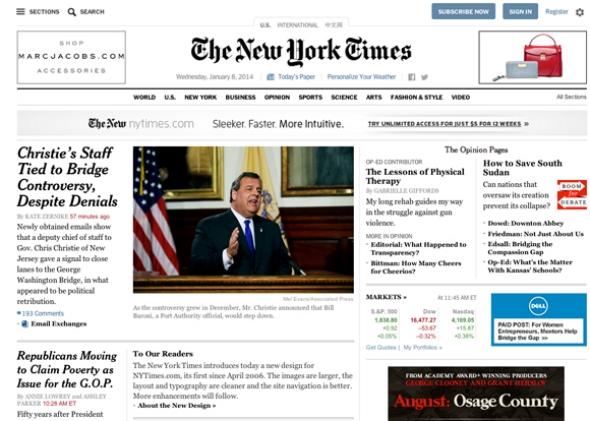The image showcases a page from the New York Times. The background is primarily white, and in the upper left corner, three lines beside the word "Sections" denote the navigation menu. Adjacent to this, a gray box advertises "shop.marcjacobs.com accessories." Beneath this, there are options for "US" and "International" editions and "The New York Times" is emblazoned in prominent black text. The date reads Wednesday, January 8, 2014. Also in the header, blue text appears for "Today's Page" and "Personalize Your Weather," with a small gray bird icon beside them. On the top right, two blue buttons labeled "Subscribe Now" and "Sign In" are present, alongside a "Register" link and a gray settings icon.

Below the header, a gray box features images of a red and a gray purse. A thick black line separates this area from the navigation bar, which includes links to World, U.S., New York, Business, Opinion, Sports, Science, Arts, Fashion & Style, and Video sections. There is a white button labeled "All Sections" in blue text.

A light blue box promotes the new NYTimes.com as "sleeker, faster, more intuitive," offering unlimited access for a minimal fee for 12 weeks. In the main content area, the headline "Christie Staff Tied to Bridge Controversy Despite Denials" is displayed prominently over a large photograph of Chris Christie sitting behind a desk with a flag and large framed pictures in the background. 

Other articles mentioned include "Republicans Moving to Claim Poverty as Issue for the GOP" and a small box addressed "To Our Readers." The right sidebar contains the Opinion section with articles such as "The Lessons of Physical Therapy" and "How to Save South Sudan," indicated by a red box with the word "Boom" alongside "Debate."

Near the bottom, a blue box discusses Dale, and a large black box at the bottom covers the film "August: Osage County."